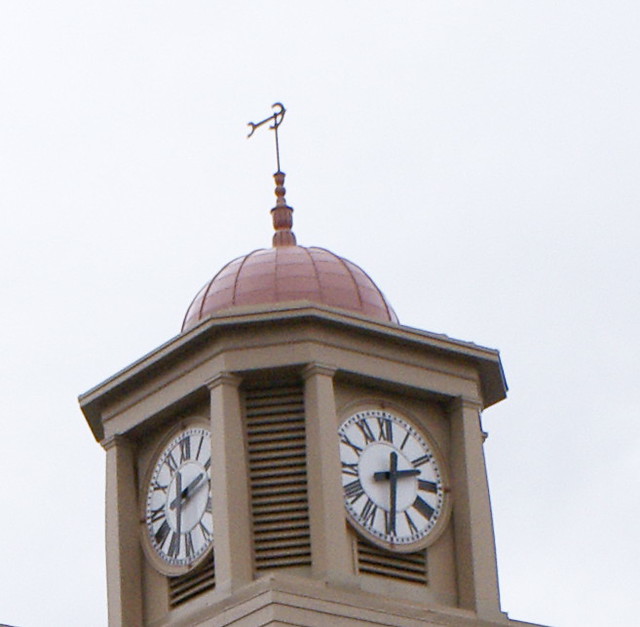This is a detailed photograph of a multifaceted clock tower, distinctly featuring two visible sides. The tower is painted a flat greenish-gray color with beige accents and is adorned with four clock faces, each depicting the time as just past 2:30 p.m. The clocks have white faces with black Roman numeral numbers and black hands, which may suggest the possibility of backlighting for nighttime visibility. At the top of the tower, there's a striking red dome from which a decorative spindle rises, leading to a wind vane that points to the right. The architectural design includes louvers and vents, enhancing its overall aesthetic and functionality. Despite the overcast sky, the tower stands out due to its attractive and detailed features.